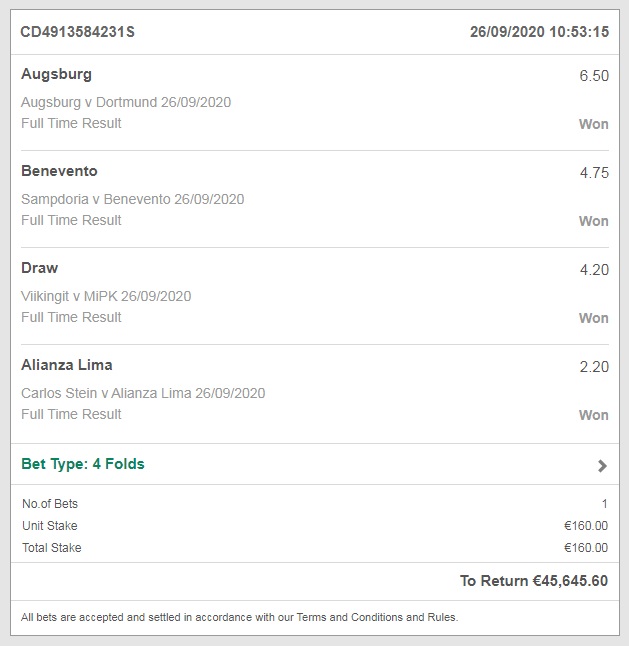Screenshot Details:

- **Reference Code**: CD49135842315 (top left corner)
- **Date and Time**: 26-09-2020, 10:53:16 (top right corner)
- **Event and Results**:
  - **Match 1**: Augsburg vs Dortmund, 26-09-2020
    - **Result**: Full-time, 6.51 WON
  - **Match 2**: Sampdoria vs Benevento, 26-09-2020
    - **Result**: Full-time, 4.75 WON
  - **Match 3**: Viking vs Mjolner, 26-09-2020
    - **Result**: Full-time, 4.21 WON
  - **Match 4**: Alianza Lima vs Carlos Stein, 26-09-2020
    - **Result**: Full-time, 2.21 WON
- **Bet Details**:
  - **Bet Type**: Four Folds
  - **Number of Bets**: 1
  - **Unit Stake**: $160
  - **Total Stake**: $160
  - **Potential Return**: $45,645.60
- **Disclaimer**: All bets are accepted and settled in accordance with our terms and conditions and rules.

This detailed caption offers a comprehensive breakdown of the betting results and conditions for full transparency.